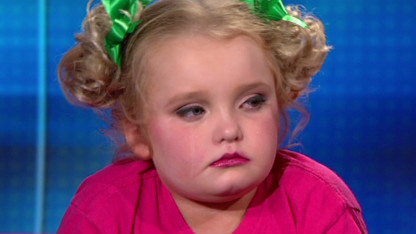In this detailed photograph, the background is a solid blue with a narrow vertical stripe running from the top to the bottom. At the center of the image stands a young blonde-haired girl with strikingly curly locks adorned by green ribbons. Her hair, styled into two perky ponytails, frames her round face. The girl's expression is serious, giving her a suspicious look as she glances sideways with her large, thickly-lashed eyes, which may be naturally voluminous or enhanced by mascara.

Her attire is a vibrant pink top with a v-neck, which contrasts sharply with the blue background. The girl's cheeks are highlighted with blush, and her lips are accentuated with lipstick, adding to her made-up appearance reminiscent of pageant participants or TV personalities like Honey Boo Boo, though it is unclear if this is actually her. In the backdrop, there is a subtle shadow hinting at a checkered pattern, blending into the monochrome blue, adding an extra layer of depth to the image.